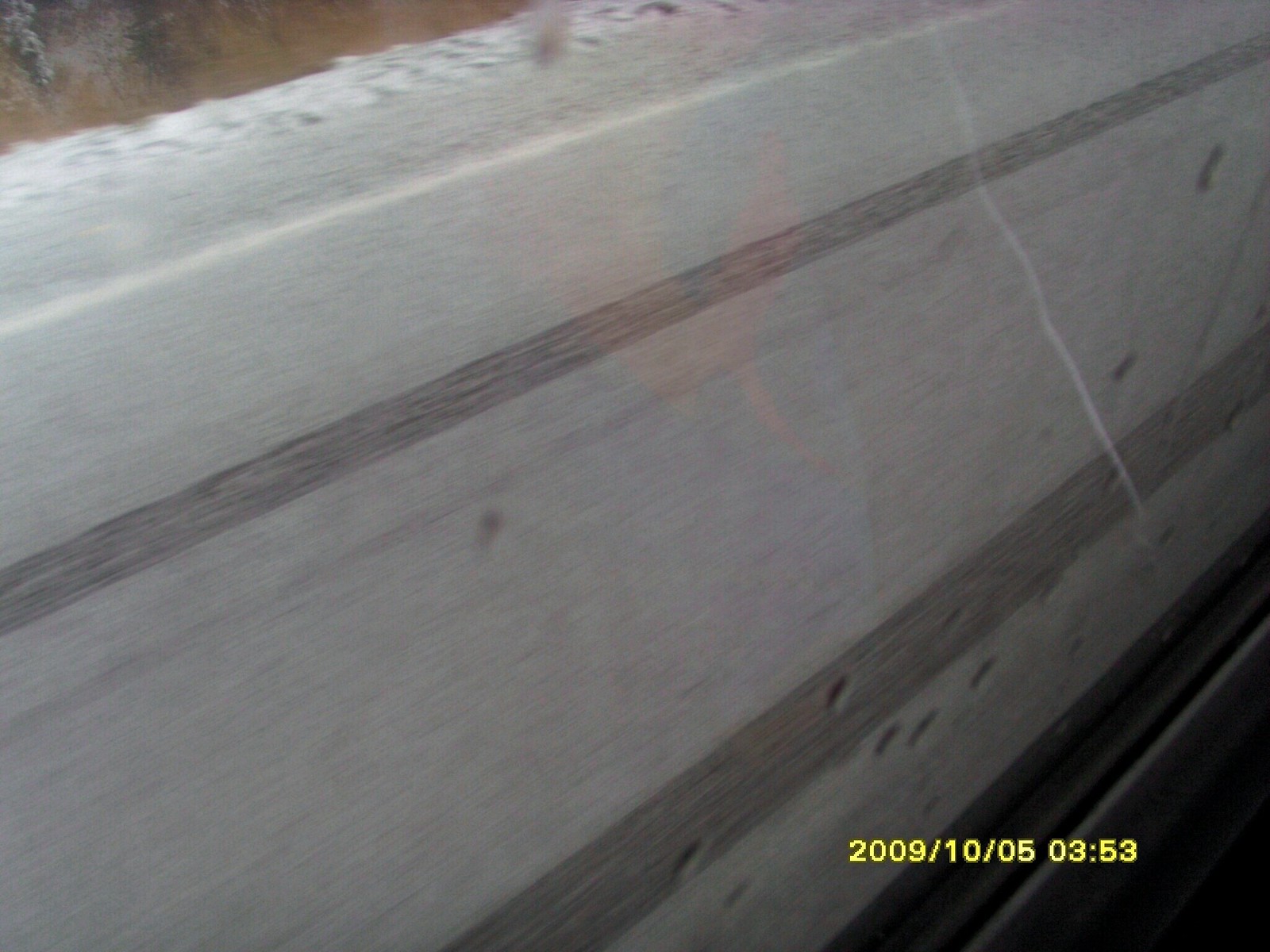This close-up photograph captures a blurred surface, suggesting movement either from the camera or the subject. In the top left corner, a medium brown triangle is visible, marred by dark gray wear. Adjacent to this is a rough, light gray area resembling concrete or stone, which transitions to a smoother texture as it extends to the right. Following this smoother section is a rounded corner that leads down to a flat, wall-like surface matching the light gray hue above. This surface is notably smooth, featuring two horizontal dark gray streaks—one smaller streak near the top and a wider streak closer to the bottom. Additionally, scattered black pock marks adorn the lower part of this surface. In the bottom right of the frame, a very dark gray triangle is present. Overlaying the image, in yellow text, is the timestamp "2009/10/05 0353."